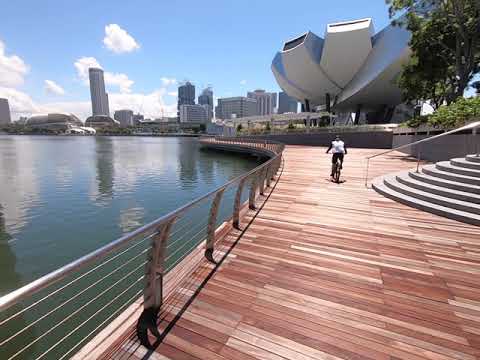The image captures a slightly out-of-focus view of a curved wooden walkway or pier along a greenish ocean adjacent to a metropolitan cityscape. The walkway itself is composed of various shades of brown planks, some even shading towards red. A person in a white shirt with black sleeves is seen riding a bicycle away from the camera along this wooden stretch. To the right of the cyclist, there's a distinct, round-shaped staircase with a shining guardrail, featuring three posts supporting it. The walkway is bordered by a silver railing consisting of a top bar held up by curved bars and interwoven with silver wires, separating it from the ocean. The water reflects the city's scattered low to medium-rise buildings, with a couple of prominent skyscrapers and a striking silver-blue structure resembling a spaceship or an art installation. The skyline extends to the upper left, showcasing a tall isolated gray tower amidst scattered clouds in a mostly blue sky. The entire scene is landscaped with intermittent plants and foliage, adding to the ambiance.